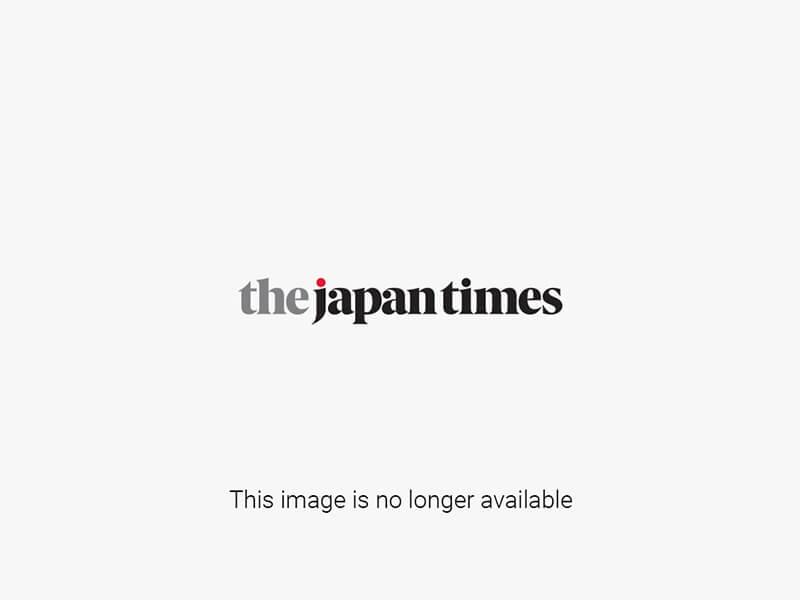This photograph features a close-up of what appears to be a sumo wrestler and a referee or judge. The sumo wrestler, centered in the image, can be seen from the chest up. He has black, pulled-back hair and is dressed in a black robe adorned with patches on the arms. He appears to be wiping his right eye with his left arm, possibly wiping away a tear or some debris from his eye. His face, although red, remains largely expressionless. Standing behind the sumo wrestler, to his right, is another man who seems to be a referee or judge. This man is dressed in a purple robe with intricate gold decorations and is wearing a black hat secured with a purple ribbon. He is holding a piece of white paper with a bit of purple fringe. The background of the image is black, making the figures and their colorful garments stand out prominently.